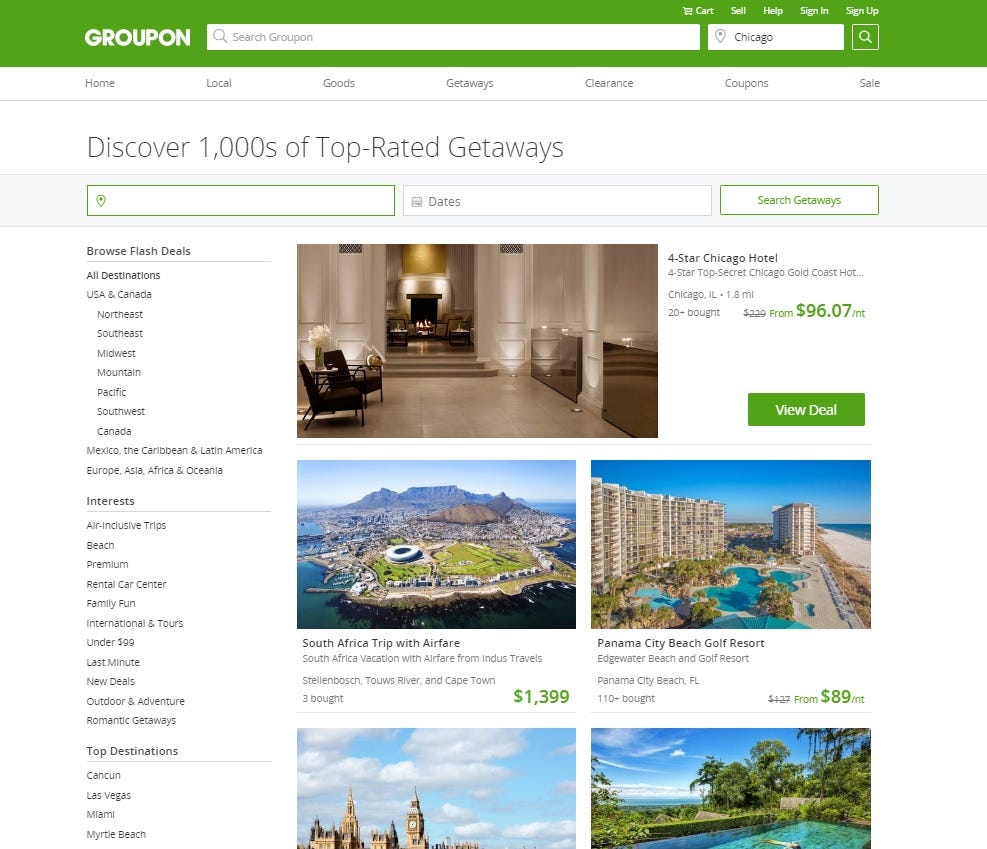The image showcases the homepage of the Groupon website, characterized by a green strip running across the top. The word "GROUPON" is prominently displayed on the left in all capital letters. Next to it is a search field labeled "Search Groupon" with the location set to Chicago. Above this area, navigation options including "Cart," "Sell," "Help," "Sign In," and "Sign Up" are visible, along with a "Search" button.

Below the main banner, the navigation menu features categories such as:

- Home
- Local
- Goods
- Getaways
- Clearance
- Groupon Coupons
- Sale

This section of the website has a white background, including the buttons. A highlighted message reads "Discover thousands of top-rated getaways," accompanied by a search bar for location and date input with a calendar icon, and a "Search Getaways" button.

On the left side of the page, a detailed navigation panel offers browsing options for various getaway deals and interests:
- Flash Deals
- All Destinations
  - US and Canada 
    - Northeast
    - Southeast
    - Midwest
    - Mountain
    - Pacific
    - Southwest 
  - Canada 
  - Mexico 
  - The Caribbean and Latin America 
  - Europe 
  - Asia 
  - Africa 
  - Oceania 

Additional categories include:
- Interest-based getaways (e.g., beach, family fun, international tours)
- Air-inclusive trips
- Premium rentals
- Last-minute deals
- Outdoor and adventure trips
- Romantic getaways 

Highlighted top destinations include Cancun, Las Vegas, Miami, and Myrtle Beach.

Centrally featured on the homepage is an enticing deal: a "Four-Star Chicago Hotel from $96.07."